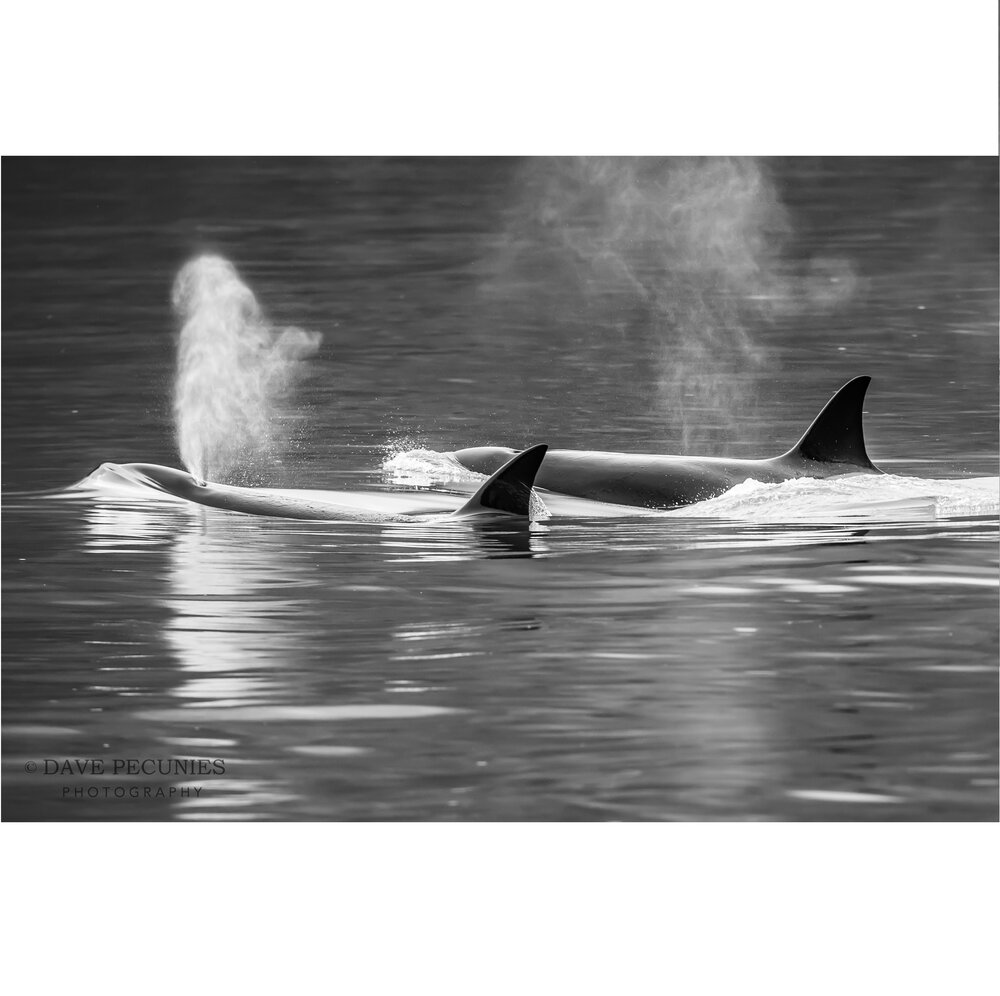The black and white photograph captures a serene moment of two dolphins breaching the calm gray waters. The dolphins are mostly submerged, with only their backs and blowholes visible. The dolphin on the left is exhaling, creating a jet or mist of air that contrasts vividly against the monochromatic background. The dolphin on the right appears to have just finished exhaling, leaving remnants of mist lingering above its back fin. Both animals display prominent triangular dorsal fins above the water's surface. In the bottom left corner, the image bears a watermark in black text reading "Copyright Dave Pucconi's Photography," indicating the artist’s authorship. The lack of color highlights the textures and details of the mist and water, emphasizing the tranquil and natural beauty of the scene. The daylight reflecting off the water suggests the picture was taken during the daytime, likely in a controlled environment given the calmness of the water.